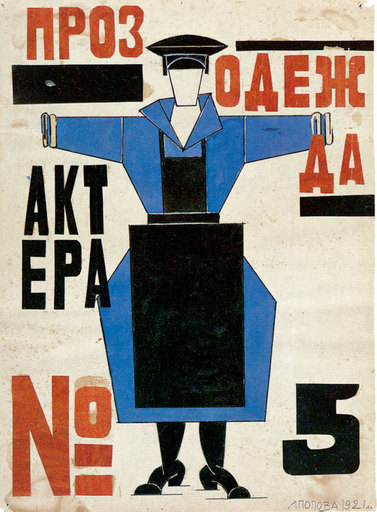The image is a color graphic illustration titled "A Female Study, Yubov Popova's Utilitarian Art" by Bogtazo, done in a constructivist style. It is a portrait-oriented poster that likely originates from an Eastern European country, as suggested by the Cyrillic writing. Central to the image is a female figure wearing a blue, below-the-knee uniform with a black apron, black stockings, and black high-heeled boots. Her arms are extended straight out to her sides. She wears a simple black hat, and her face is without any discernible features. The overall composition is characterized by shapes — squares and rectangles dominate the design. The background is white, featuring multiple pieces of text: "NPO3" and "0AE" in the upper section, "AKTEPA" in the upper left, "A-K-T-E-P-A" in black on the left arm, "N-O" with an equal sign beneath the "O" on the lower left, and the number "5" to the lower right. There are also two small rectangles within the background.